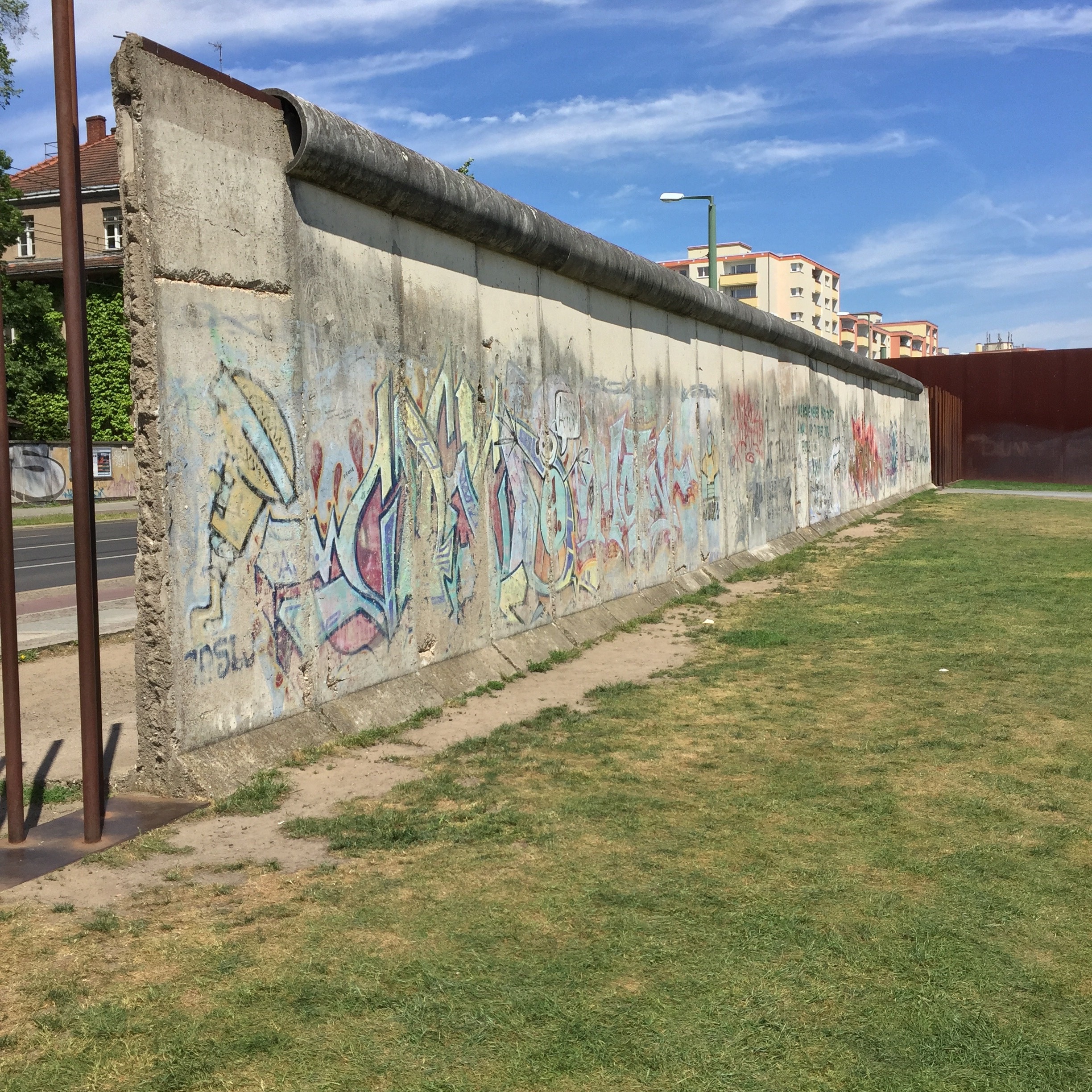This photograph captures an outdoor urban scene centered on an old concrete wall adorned with faded graffiti in a multitude of colors, including yellow, blue, red, and green. The graffiti sprawls across the entirety of the wall, although much of it is indistinct due to weathering and possible overpainting. The wall, light gray and somewhat deteriorated, slants from the left side of the image to the right, making the right end appear smaller. At the top of the wall runs a black pipe, and to the far right, a tall wooden brown fence extends upward. 

In the foreground, patchy, sparse grass interspersed with sections of dirt extends to the lower right of the image, indicating a neglected or abandoned yard. Two rusty metal poles are positioned in front of the wall. Behind the wall, a street is visible along the left edge, bordered by tall residential buildings of light beige or yellowish color with hints of orange trim, likely apartment complexes. 

Streetlights and some silhouetted house structures shaded by trees also appear in the background. The sky is clear and blue, with only a few wispy, brilliant white clouds, suggesting a sunny day.